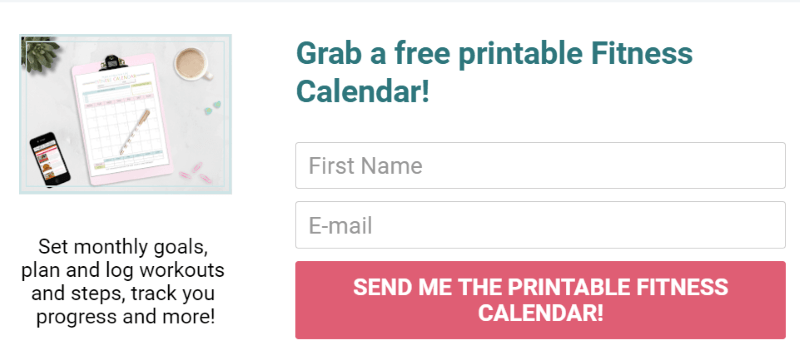Title: "Grab a Free Printable Fitness Calendar!"

The image features an advertisement for a free printable fitness calendar. At the top of the image, there's a bold, inviting headline that reads, "Grab a Free Printable Fitness Calendar!" Below this headline is a form, prominently displayed.

The form consists of several rectangular input fields:
1. **First name** – The first rectangle prompts users to enter their first name.
2. **Email** – The second rectangle is for users to input their email address.

Beneath these fields is a reddish-pink rectangular button with white text that says, "Send me the printable fitness calendar!"

To the left of the form, there is an image of a calendar against a light purple background. The calendar image is elaborately styled with several elements:
- A cup of coffee is positioned at the top right corner.
- To the top left, there appears to be a partial house plan sketch.
- At the bottom left, there’s a black cell phone.

Underneath the calendar image, a detailed caption in black writing outlines the benefits of the calendar:
- "Set monthly goals."
- "Plan and log workouts and steps."
- "Track your progress and more!"

The entire advertisement is set against a white background, with a very thin horizontal gray line at the top acting as a sleek boundary for the image. This clean and organized design invites users to easily sign up for the helpful fitness resource.